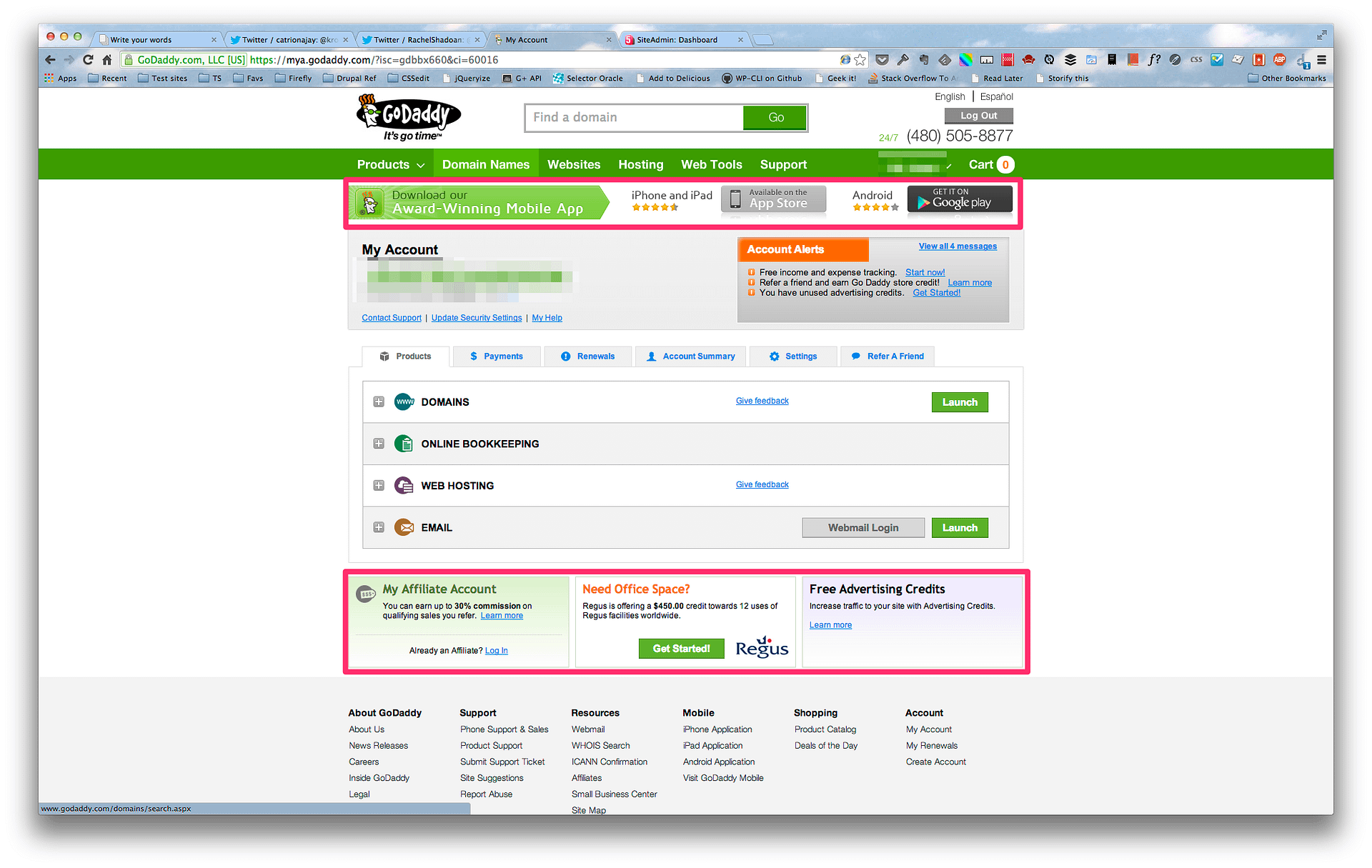This detailed screenshot captures a full view of a desktop browser navigating the GoDaddy.com website. The browser's URL bar at the top prominently displays "godaddy.com, LLC" alongside a green lock icon and green text, indicating a secure connection. The website's design features a blue sky and cloud motif at the top.

The layout exhibits substantial empty white space on both the left and right sides, with the primary content centered on the page. Two specific ad banners are the focal points, each highlighted with red boxes to emphasize their significance.

The first highlighted banner, positioned near the top of the page, advertises GoDaddy's award-winning mobile app and includes icons for the Google Play Store and the App Store.

The second highlighted banner, located near the bottom, is divided into three parts. The left section reads "My Affiliate Account," the middle part states "Need Office Space Regis," and the right section promotes "Free Advertising Credits."

Overall, the screenshot effectively draws attention to the advertised services while showcasing GoDaddy's secure and user-friendly website layout.